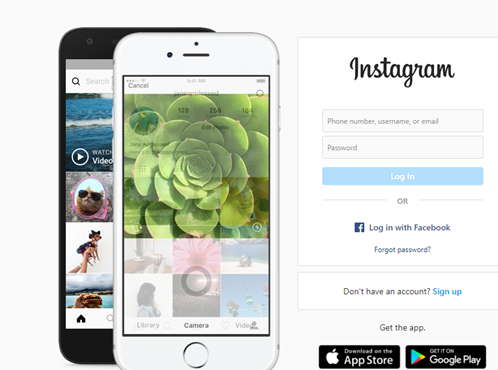On the left side of the image, there are two cell phone screens displayed. The phone in the background, predominantly black, shows only its right half. Its screen displays an ocean image with a circle icon and an arrow indicating a 'watch video' option. Below that, there's an image of a cat wearing sunglasses and a blue hat, followed by a picture of a dog dressed in a costume. The last image on this phone screen is of a bright blue ocean with clouds in the sky.

To the right, a slightly blurry white cell phone is visible. Its screen shows a green plant with detailed petals. At the bottom of this screen, there are three options: 'Library', 'Camera', and 'Video'.

On the far right, the Instagram login section is displayed. The word "Instagram" is written in black cursive text. Below this, there are fields to input a phone number, username, or email, along with a password field. A long blue rectangle below these fields serves as the 'Log In' button. Additional options include logging in with Facebook, a 'Forgot password?' link, and a 'Don't have an account? Sign up' link in blue text.

At the bottom, there are download options: one for the App Store, indicated by a white apple icon, and another for Google Play, represented by a right-pointing triangle with blue, pink, and yellow colors.